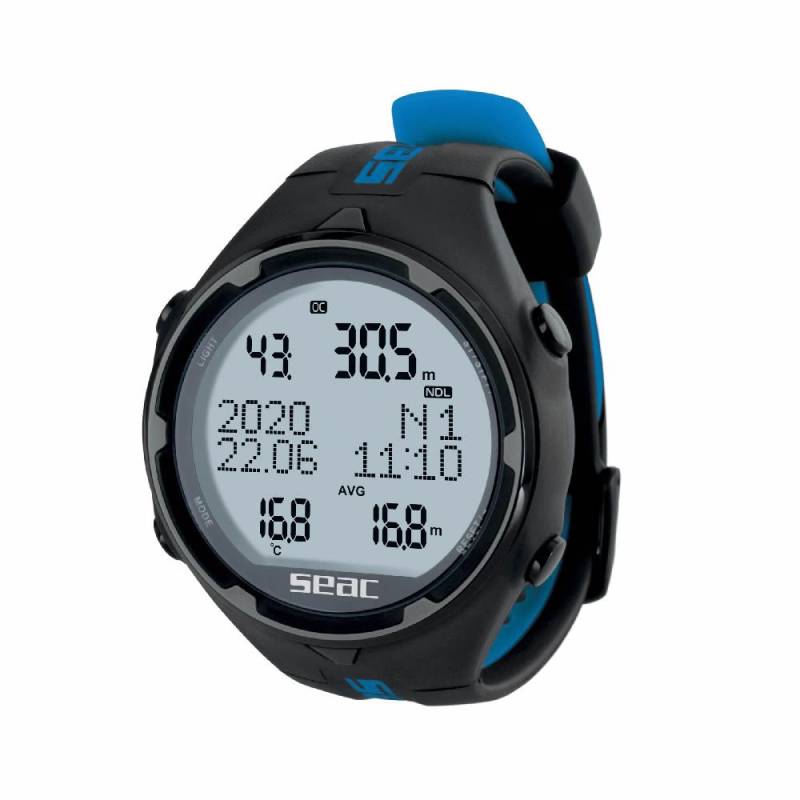The image features a detailed close-up of a smart watch with a predominantly black exterior and subtle blue accents on the inner side of its wristband and near the fastening area. The watch face itself is round and encased in a black rubber-like outer rim with a gray border around the center. The display background is light gray, showcasing an organized array of numerical data. At the bottom of the watch face, the brand name "SEAC" is prominently displayed in white uppercase letters. The top portion of the display reads "CC" in black text and two columns of information are visible. The left column includes "43", the date "2020-22.06", and "16.8C" indicating the temperature. The right column displays "30.5 meters," followed by "N1" and "11:10," which likely represents the current time, and the average depth "16.8 meters." Additionally, the watch features small round buttons on both sides, partially visible near the top and bottom. The background of the image is a plain white, highlighting the watch without any distractions.